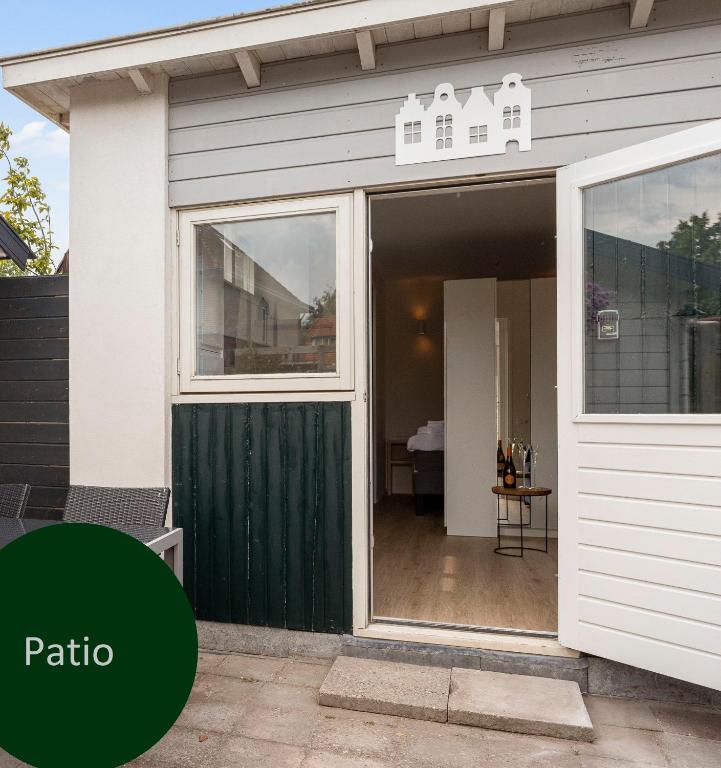This detailed daytime photograph captures the exterior of a charming single-story cottage-style home with gray and white aluminum siding. The image is taken from outside the house, focusing on the patio area. To the left, two brown patio chairs and a table are visible, with a brown wooden fence in the background. The ground is paved with gray, stone-like bricks, creating a neat patio surface. A green circular icon with the white text "patio" is digitally added to the lower-left corner, hinting at an advertisement. 

The house features a door on the right side that is wide open, half composed of glass and half wood, offering a clear view into the cozy interior. Inside, there's a small table set with wine bottles and glasses, located on a wooden floor. Above the doorway, a small decorative accent resembling white miniature houses adds charm to the scene. A glass window on the left side of the house complements the inviting entryway. The sky is clear and blue, and a small tree is visible in the background, enhancing the overall inviting atmosphere of this picture-perfect patio setting.